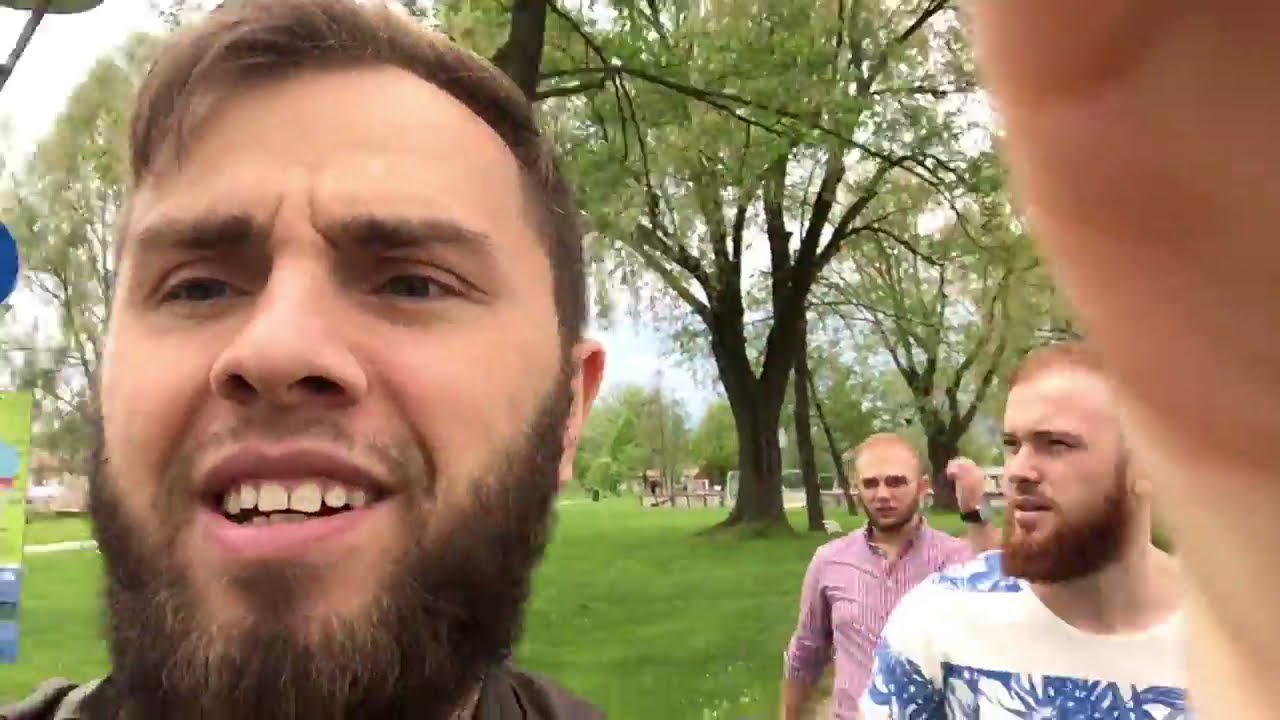The image captures an outdoor scene set in a public park or similar green area, likely during the middle of the day given the bright but cloudy sky. In the foreground on the bottom left of the image, a man with short wavy brown hair, a black beard, and partial mustache looks directly at the camera. He's positioned from the neck up, his shoulders just visible, and is wearing a dark purplish-brown shirt. His mouth is slightly open, and he has brown eyes. 

To the bottom right of the image, another man is present. This man, appearing waist-up, also has short brown hair along with a beard and mustache. He wears a white shirt featuring a blue floral stripe and holds a phone in his right hand, partially blocking the camera. 

Behind these men extends a grassy area dotted with trees. Just over the shoulder of the man on the right is a prominent tree, while a line of more trees along a walking path trails off further into the background. A building with a reddish roof can be seen in the distance amidst the greenery. Additionally, there is a table on the far side of the grassy area and what appears to be a soccer goal even further back, completing the detailed setting of this lively outdoor environment.